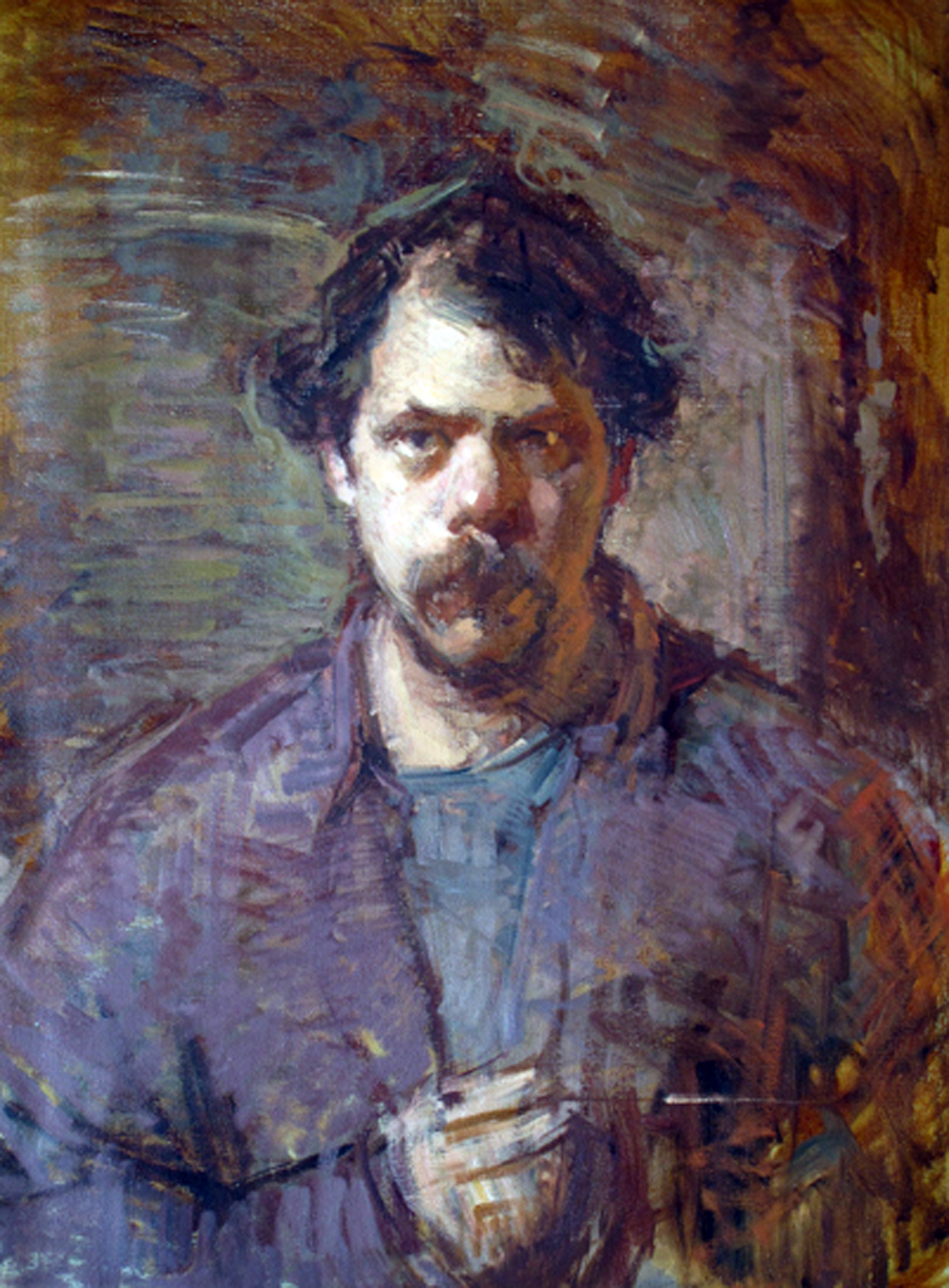This impressionist painting captures a man with hurried and dynamic brushstrokes, characteristic of the style. The man has prominent tufts of black hair contrasting with his shiny, light-colored forehead. His nose is notably large and tinged with a pink beige hue. Adding to his distinctive features, he sports a gray beard and mustache. He is dressed in a dark purple shirt with a collar, over a blue undershirt. His right hand is partially visible over his chest. The background features broad brown brushstrokes, particularly concentrated in the top right corner, providing a rustic frame to the composition.